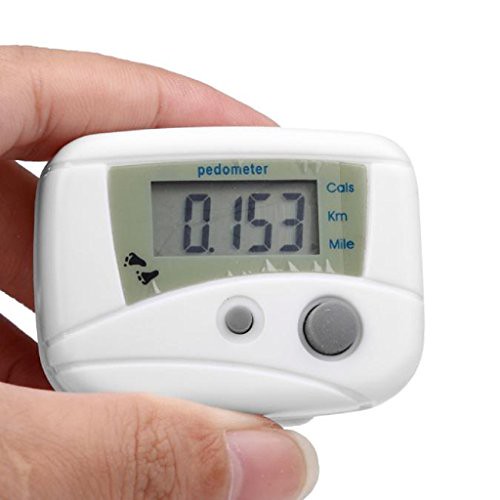This is a high-resolution color photograph featuring a handheld white pedometer against a stark white background. The pedometer is firmly grasped between the thumb and forefinger of a hand with relatively long, unpainted nails, though the rest of the hand is not visible.

The top of the pedometer is labeled with the word "pedometer" in lowercase blue letters. To its right, there are indicators reading "CALS," "KM," and "mile," accompanied by a small screen display. The screen currently shows the number "0.153" with a caret symbol next to "mile," signifying the device is set to measure miles.

At the bottom left of the pedometer, two small black footprints are printed, adding a touch of design. The control interface includes two circular buttons: a smaller gray one in the center and a larger gray one on the right. Close inspection of the screen area reveals a slightly wrinkled plastic protective layer, which appears a bit cut off, adding a touch of imperfection to the device's otherwise sleek appearance.